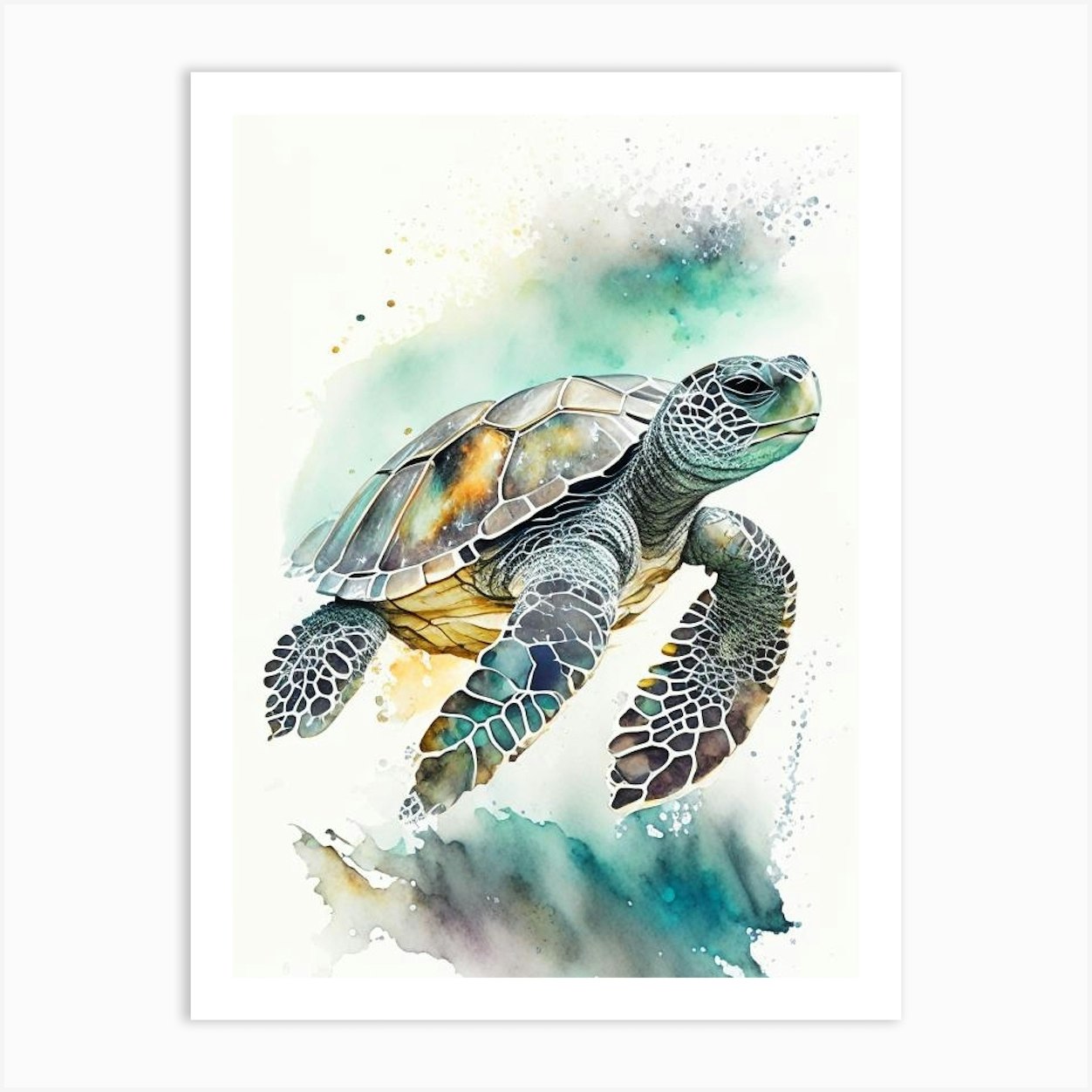The image depicts a detailed, vibrant representation of a sea turtle, which appears to be created using a combination of watercolor effects and possibly digital techniques. The orientation is portrait, set against a plain white background. The sea turtle, positioned centrally, is swimming rightward at an upwards angle, with its head on the right and tail on the left. 

Its distinct flippers are down, with the right one extending out and downward and the left one curving inward to the right before dipping back down. The turtle's underbelly shows hues of yellow, while its shell features a mix of light gray, green, purple, and yellow tones, adding to the depth and realism. Notably, the turtle's flippers and parts of its body exhibit blue, green, and purple splashes, enhancing the vibrant lifelike feel. Around the turtle, there are watercolor-like splashes in shades of green, purple, blue, gray, and black, particularly evident at the top and bottom of the image, giving the composition an artistic, fluid effect. The turtle seems to be gazing towards the viewer with a closed mouth, adding a sense of interaction and intrigue to the image.